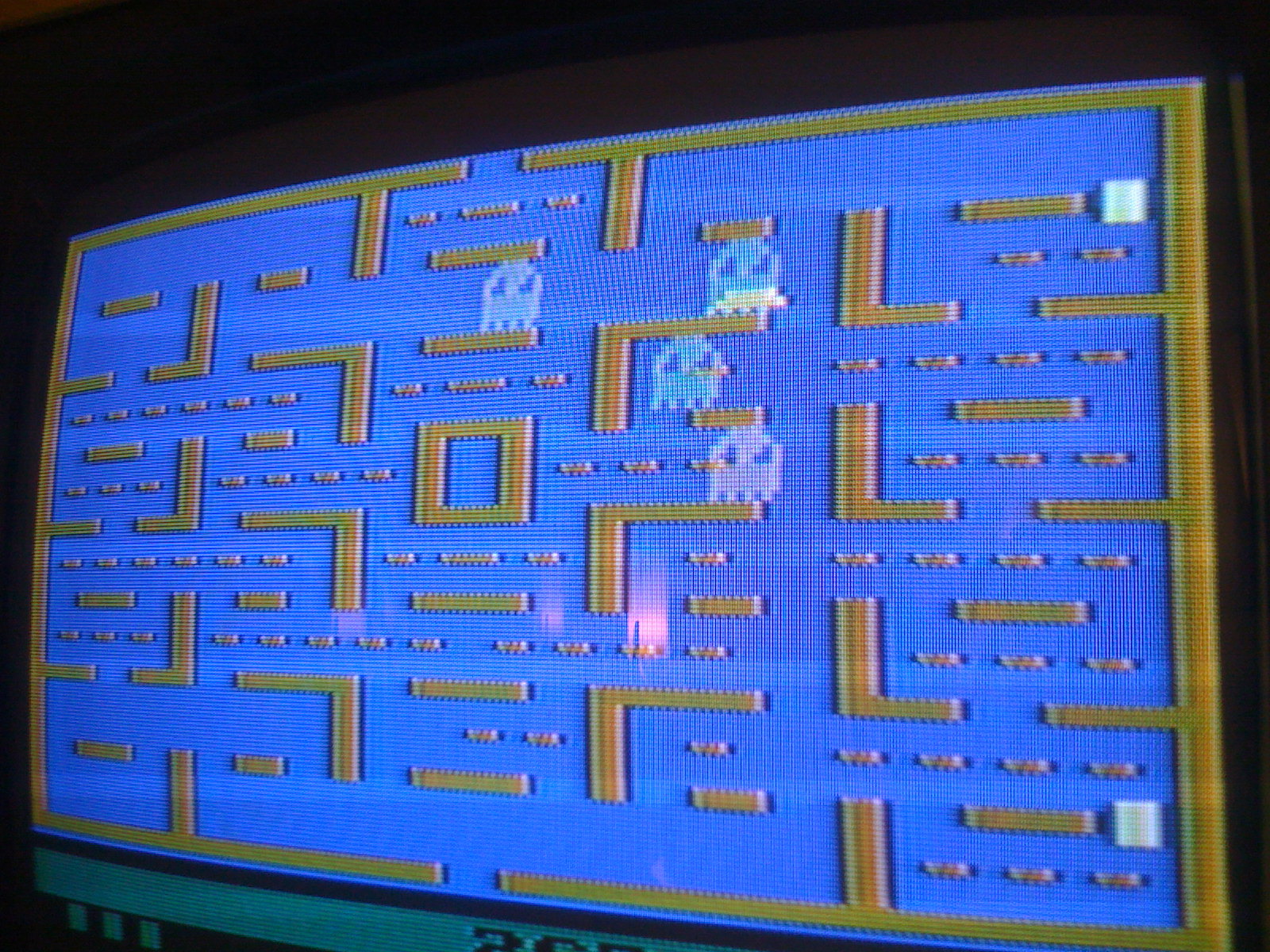This detailed color photograph captures a widescreen TV displaying a scene from the Pac-Man video game. The screen has a blue background, showcasing the iconic maze constructed from numerous geometric shapes. Notably, the four ghosts within the maze are all blue, indicating that Pac-Man has recently consumed a power pellet, although Pac-Man himself is not visible in the frame. The graphics are distinctly blocky, suggesting this is potentially the Atari 2600 version of the game, rather than the more refined graphics of the arcade edition. The image is devoid of any text, people, animals, or plant life, focusing entirely on the nostalgic gaming experience.